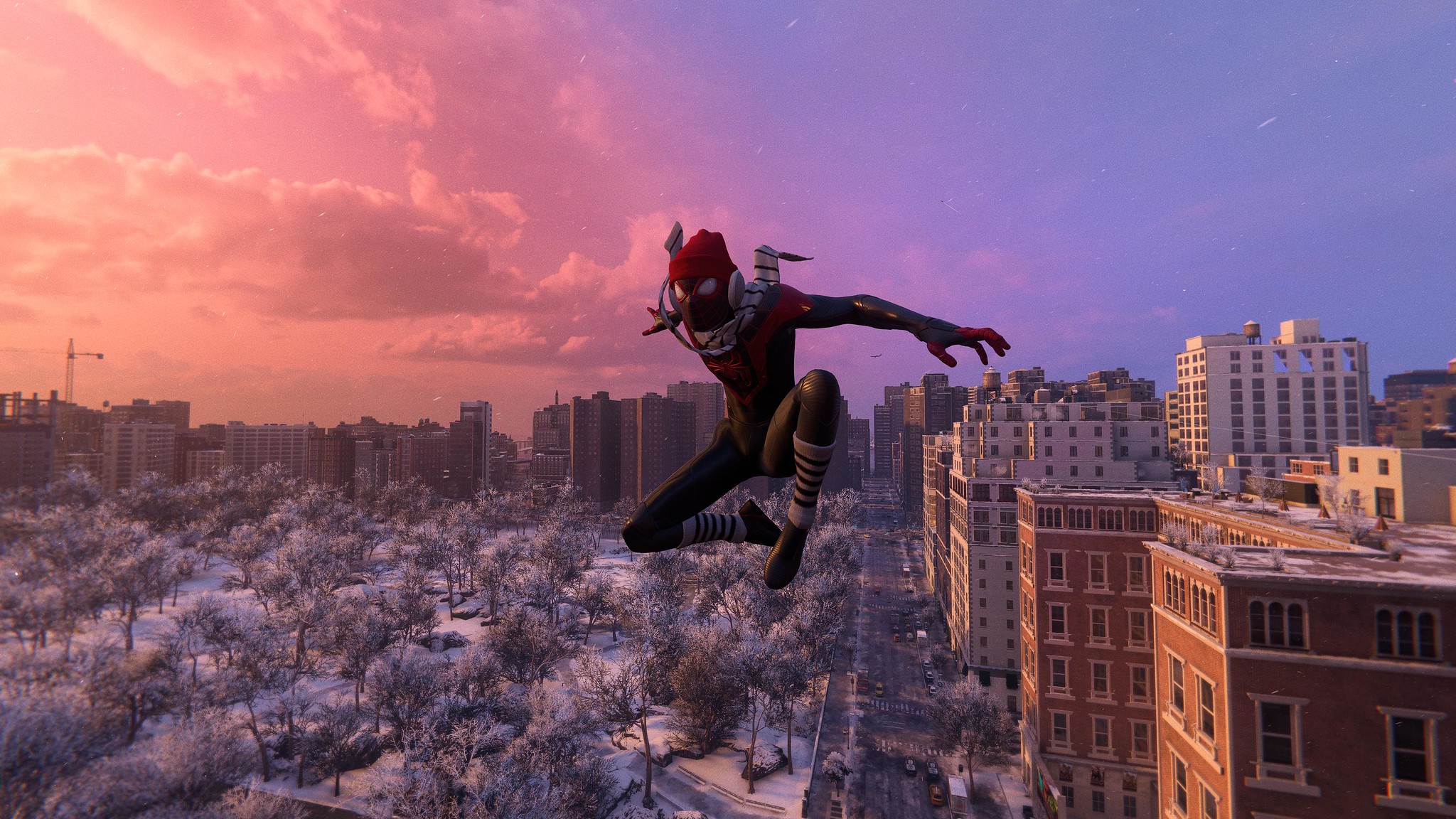A computer-generated image depicts a dynamic scene reminiscent of a Spider-Man character. The figure is clad in a predominantly black, skin-tight suit accented with red around the chest and red fingertips. He accessorizes with a striking red hat and a gray and white scarf, and knee socks are visible beneath the suit. The backdrop is a snow-covered urban landscape, evoking the ambiance of a place similar to Central Park, surrounded by towering skyscrapers and various apartment buildings. A wide, bustling residential street with four or five lanes runs through the scene on the center right. The character is captured in mid-leap, with arms outstretched like claws, one leg raised and the other bent underneath him, against the backdrop of a sky illuminated by a setting or rising sun. The overall effect is both dramatic and atmospheric, emphasizing the contrast between the dark attire and the bright, snowy environment.